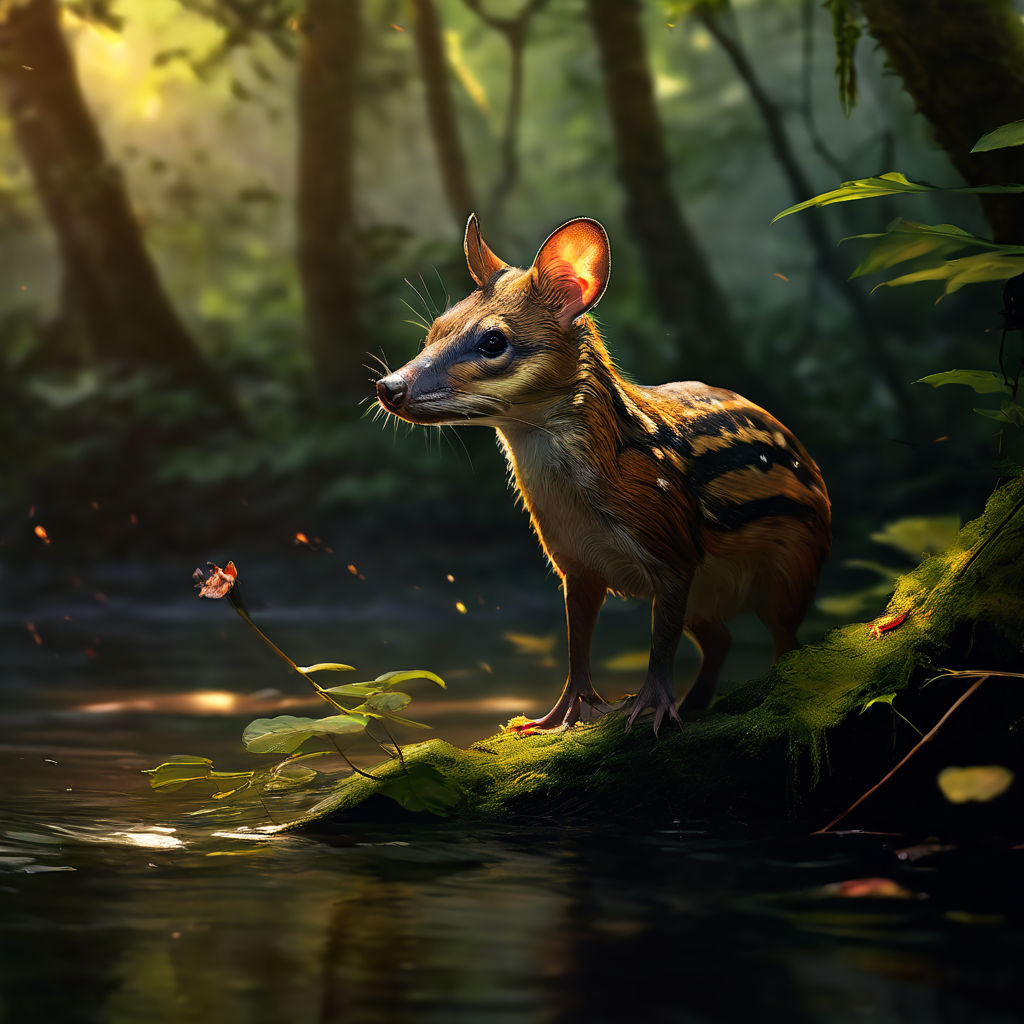In the middle of a dense, sunlit forest, a small, mouse-like marsupial stands on its hind legs atop a moss-covered tree root near the edge of a tranquil creek. This cute creature, not quite a mouse, features big, round ears that glow orange in the sunlight and a long snout adorned with whiskers. Its fur is primarily brown with black stripes across its back, accented by a few white flecks. The marsupial’s forearms, ending in five clawed paws, are slightly lifted off the ground as it gazes to the left. The vibrant green moss beneath, coupled with the light filtering through the canopy, highlights its striking coat of mixed red, gold, orange, yellow, and white hues, making the scene both serene and picturesque.